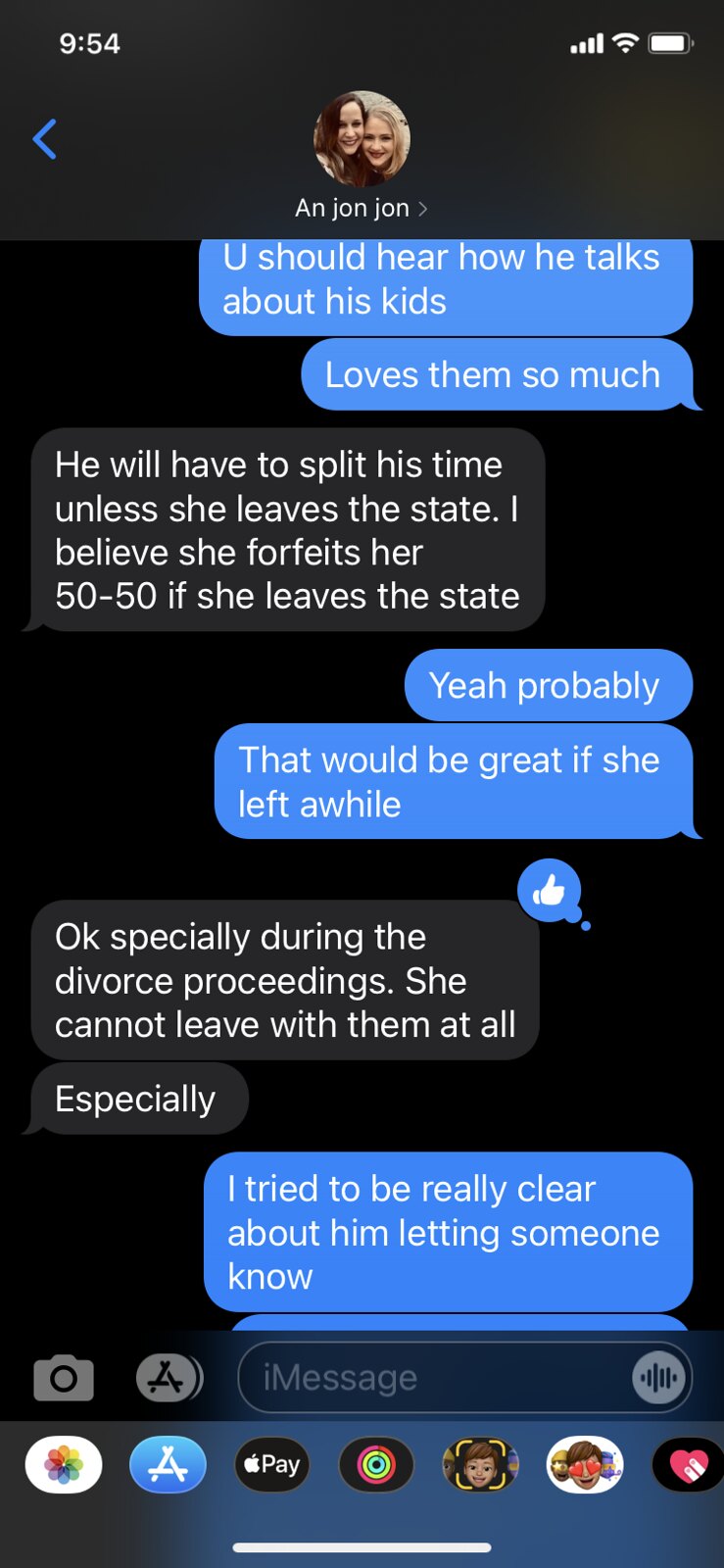A screenshot of an iPhone text message conversation at 9:54 shows the typical cellular details: a nearly full battery, phone signal, and Wi-Fi signal. The image features a circular profile photo of two smiling young women, one with dark hair and the other blonde. The conversation is between the user and someone named Ann JohnJohn. The first message reads, "You should hear how he talks about his kids, loves them so much." The reply, in a gray background with white text, states, "He will have to split his time unless she leaves the state. I believe she forfeits her 50-50 if she leaves the state." This is followed by a blue response, "Yeah probably, that would be great if she left a while," accompanied by a thumbs-up emoji. Another gray message says, "Okay, especially during the divorce proceedings, she cannot leave with them at all especially." Finally, a blue message reads, "I try to be really clear about him letting someone know." Below the conversation, typical iPhone elements are visible, including the camera icon, the "A" for apps, and icons for Apple-related features like iMessage, Apple Pay, and photo sharing.